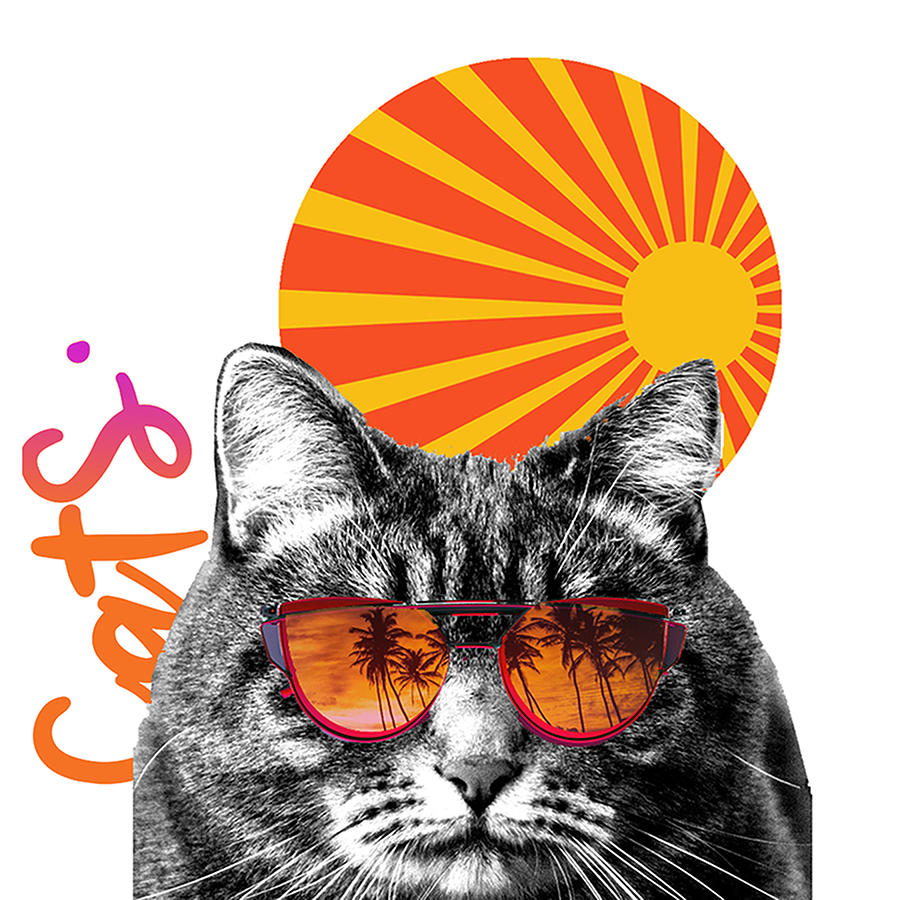This is a digitally created, surreal poster featuring a black and white cat, potentially a Maine Coon, with an 'M' marking on its forehead. The cat sports rimless, orange sunglasses that reflect a picturesque sunset and palm trees. Its facial expression is neutral and calm. The background is stark white, enhancing the contrast with the colored elements. To the left of the cat in vertical, cursive text is the word "cats," displayed in an orange to purple gradient. Behind the cat is a radiant sun illustration, composed of a central orange circle with patterned, parallel yellow rays extending outward. A smaller yellow circle is positioned to the right of the larger sun graphic. The overall composition creates a vibrant, playful atmosphere with a blend of black-and-white and colorful graphics.